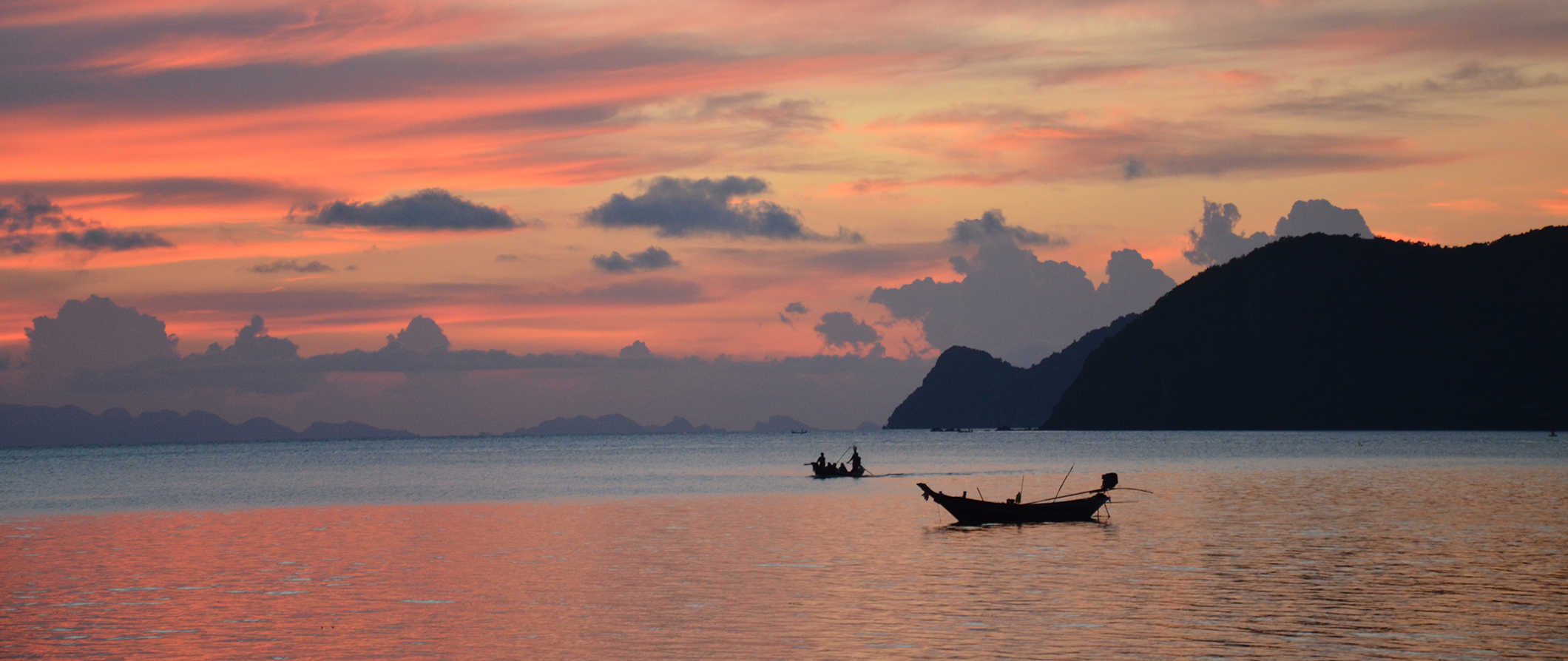This panoramic color photograph captures a tranquil bay or large lake at sunset, rendered in a photographic representational realism style. In the foreground, a small, empty sailboat or rowboat floats serenely on the water's still surface, which mirrors the dramatic sky above. Further out, another boat, possibly a fishing boat of Asian style, has a few indistinct figures standing, appearing tiny against the expansive landscape. On the right, a prominent mountain formation rises sharply from the water, its silhouette a deep, almost black shade of blue. The far horizon is lined with distant mountains shrouded in low clouds, with the sky awash in the warm, glowing hues of dusk. Puffy clouds tinged pink and purple add depth and texture, their reflection casting a matching glow on the water below, creating a harmonious and serene scene.